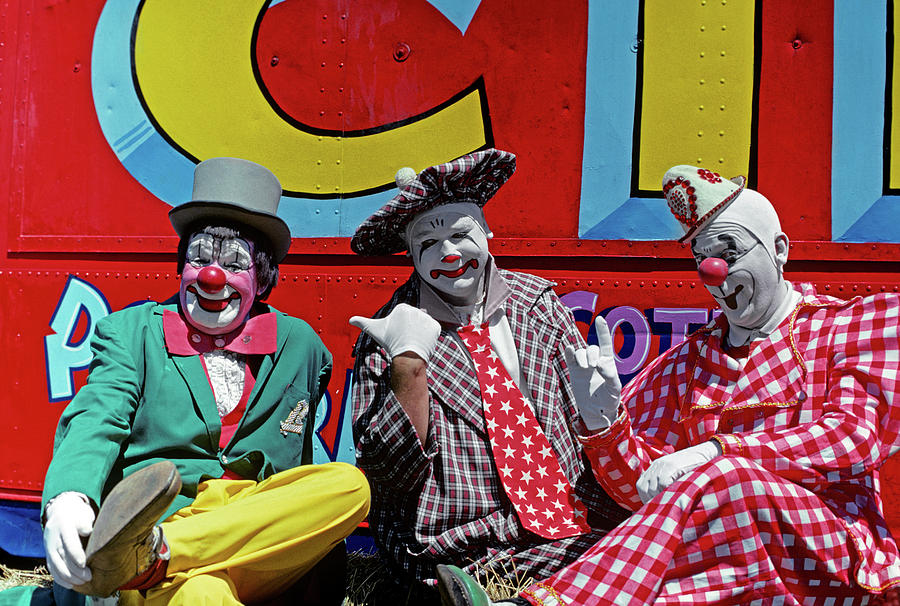The photograph, taken outdoors during a sunny daytime, features three men dressed as clowns sitting in front of a large red railway car. The railway car has yellow lettering with black outlines and blue highlights that spell out "CIRCUS." The vibrant sign boasts a 3D effect and sits prominently above the clowns. 

On the left, the first clown dons a gray top hat, has a large red bulbous nose, black hair, and reddish cheeks and chin. His face is predominantly white with black and white detailing around the eyes. He wears a green dress jacket, red shirt over a ruffled white shirt, yellow pants, oversized black shoes, white gloves, and a large flat red or pink bow tie. His attire is slightly tattered, and he has his arm behind his back.

The middle clown sports a red, white, and black checkered flat hat and a matching suit. His face is white with red paint on his nose and around his lips, sans pink. He has white gloves and a red necktie adorned with white stars. He stands out with his thumb jutted out, as if hitchhiking.

On the right, the third clown wears a small white hat with red beads that barely fits his head and a white bald cap. His face is painted white with a large red nose. He wears a red and white checkered uniform, white gloves, and has his hand up with his thumb touching his middle and ring fingers, while his index and pinky fingers are extended, like a rock sign. His legs are crossed as he sits.

The strikingly colorful and exaggerated outfits, make-up, and comical hats of the clowns contrast vividly against the bold red backdrop of the circus railway car, making for a lively and engaging scene.